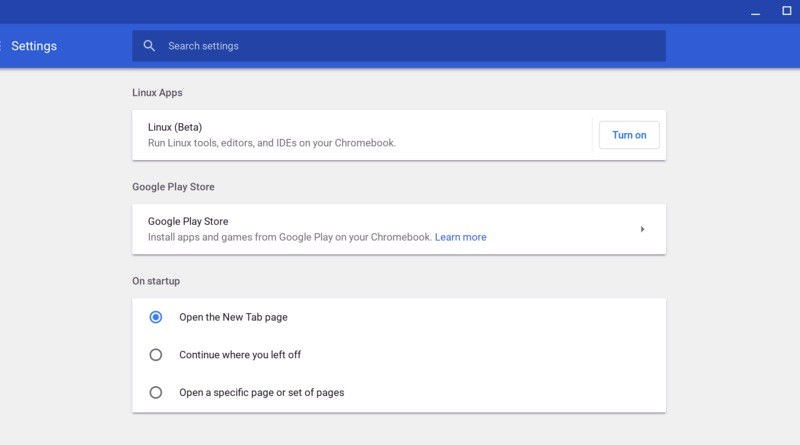The image shows a screenshot of a computer settings window. The screen is significantly wider than it is tall, and features a distinct layout with multiple sections and banners.

At the very top is a dark blue banner with standard window control buttons on the right (minimize, maximize, and close). Directly below this is a slightly lighter blue banner, which spans the width of the screen. On the far left of this banner, the word "Settings" is prominently displayed in white text. More centrally located on this banner is a dark blue search bar labeled "Search settings," allowing users to type and search for specific settings.

The main content of the screen, under the blue banners, sits on a gray background. At the top of this section, in bold black letters, we see the heading "Linux apps." Just beneath this heading is a light grayish bar with the subtitle "Linux (Beta)" in parentheses.

Below the subtitle, a description reads: "Run Linux tools, editors, and IDEs on your Chromebook." To the right of this text, there is a button labeled "Turn On," presumably to activate the Linux (Beta) feature.

Further down, another section is titled "Google Play Store," accompanied by a similar white bar. This section includes a description: "Install apps and games from Google Play. Learn more." To the right of this description, there is an arrow button signifying further options or information.

At the bottom of the screen, the "On startup" section is outlined within a taller white rectangular box, divided into three radio-button options. The first option, which is pre-selected with a blue dot, is labeled "Open the New Tab page." The second option states "Continue where you left off." The final option reads "Open a specific page or set of pages," allowing users to configure their startup preferences.

Overall, the screenshot captures a detailed view of a settings interface, showcasing available options related to Linux apps, the Google Play Store, and startup behavior.